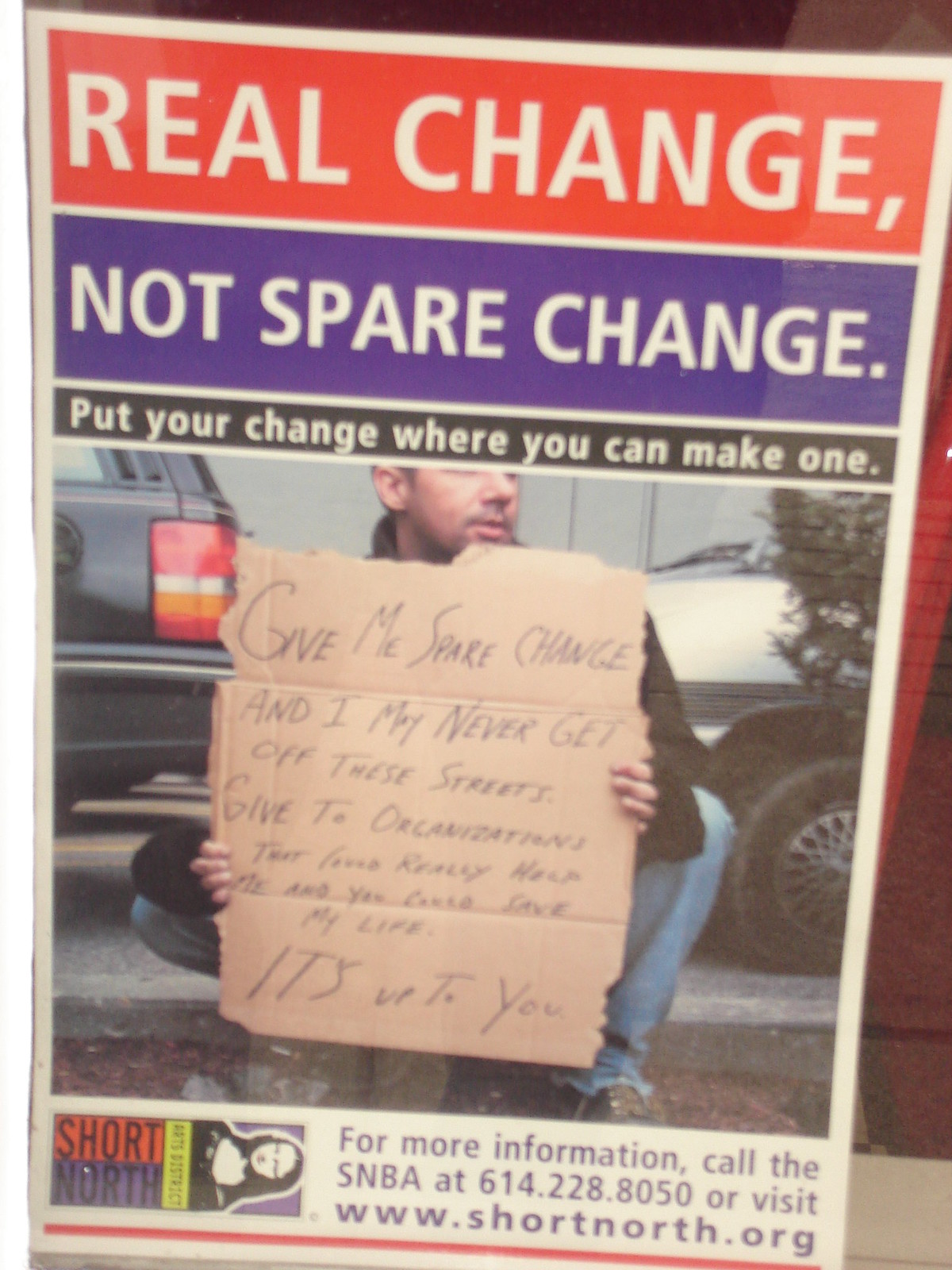The image is a striking advertisement consisting of three text banners with a compelling visual and contact information below. At the top of the poster, there's a prominent red text box with a red background and white text that reads, "REAL CHANGE," all in capital letters. Following this, a blue text box with white text says, "NOT SPARE CHANGE." Below that, a black text box with white text declares, "PUT YOUR CHANGE WHERE YOU CAN MAKE ONE."

In the center of the image, there is a poignant scene featuring a man kneeling on the ground. He is dressed in blue jeans and a black sweatshirt, with only the lower half of his head visible due to the upper part being cut off by the frame. He is holding a cardboard sign that partially reads, "Give me spare change, and I may never get off these streets. Give to organizations that really help and you could save my life. It's up to you." This message is slightly blurred, making it challenging to capture every word. Behind the man, a black car faces left, and behind it, a gray car is partially visible, showing just the rear end.

At the bottom of the poster, there is a note indicating, "Short North," alongside a sideways image of the Mona Lisa. For more details, the poster provides contact information: "For more information, call the SNBA at 614-228-8050 or visit www.shortnorth.org."